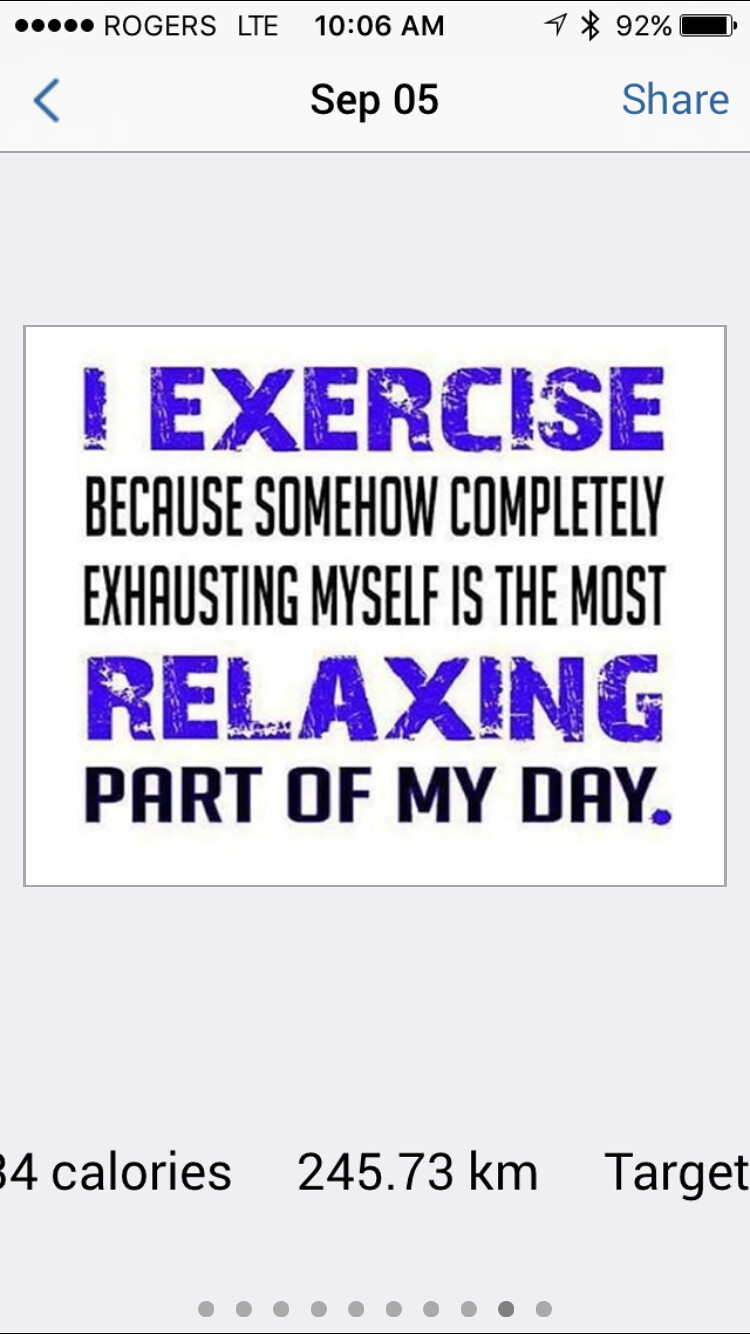The image is a vertically oriented screenshot or photograph of a smartphone screen, exhibiting a light gray background. At the top, it's outlined by a gray header with pinstripe black borders at the top and bottom. In the upper left-hand corner, five small black-filled circles are aligned horizontally. Next to these, in black text, it reads "Rogers LTE 10:06 AM." Adjacent to this are icons indicating Bluetooth connectivity and a battery level at 92%.

Below this header on the left-hand side is a blue left-pointing arrow, while in the center, the date "September 05" is displayed. To the right, the word "Share" appears in blue.

The central focus of the image is a square with a thin outline on a white background. It contains a motivational meme that reads:

"I exercise" (in purple)
"because somehow completely exhausting myself is the most relaxing part of my day." 

Here, "relaxing" (in purple), and "part of my day." (in black) are distinctly highlighted with a purple period at the end. Below this text, the screen shows clipped information that reveals partial data: an 8 and a 4 indicating calories, followed by "245.73 KM" and to the right, the word "target." 

At the very bottom center of the image, there are 10 small gray circles, commonly associated with swipe navigation in apps like Instagram, where this appears to be the second images from the end.